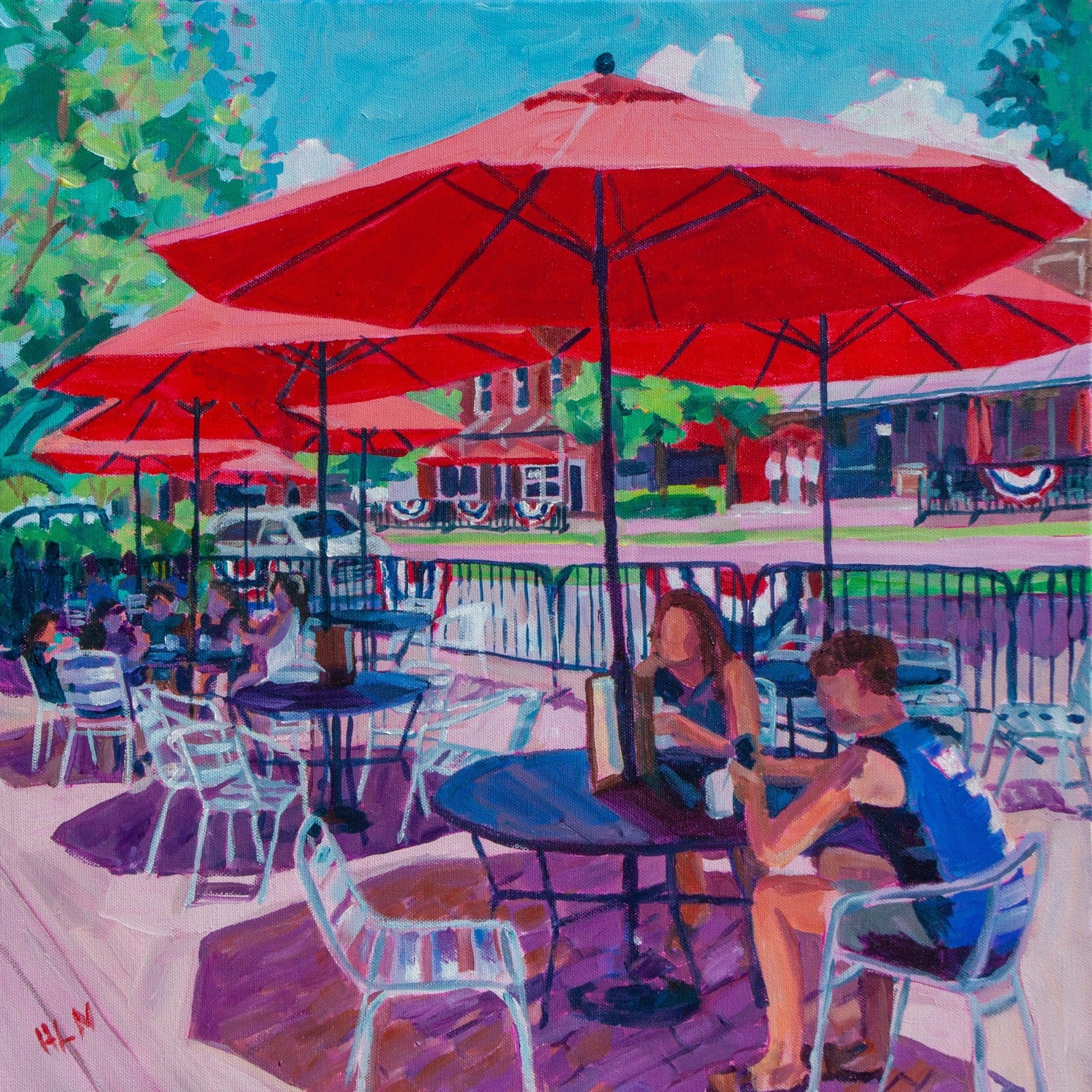The painting depicts an outdoor dining area, likely part of a restaurant during a daytime event. It prominently features two people sitting at a round black table with a large red umbrella providing shade through its center. The man, faceless, is dressed in a blue tank top, gray shorts, and flip-flops, and is engrossed in his phone while sitting on a simple white metal chair. Across from him is a woman, also faceless, who appears to be wearing a dark blue or possibly purple dress. The surrounding area is filled with identical tables and white chairs, some of which are occupied by other patrons, including a family. Others remain empty. Beyond the dining area, there's fencing adorned with red, white, and blue banners, suggesting the setting is part of a larger event. Cars are parked around the fenced area, and buildings with similar decorations are visible in the distance, with groups of people gathered in front of shops. The painting is rendered in various hues of green, red, and blue, and includes the initials "HLM" in red in the bottom left corner. The backdrop features more tables, trees, and a blue sky, enhancing the lively, communal atmosphere of the scene.